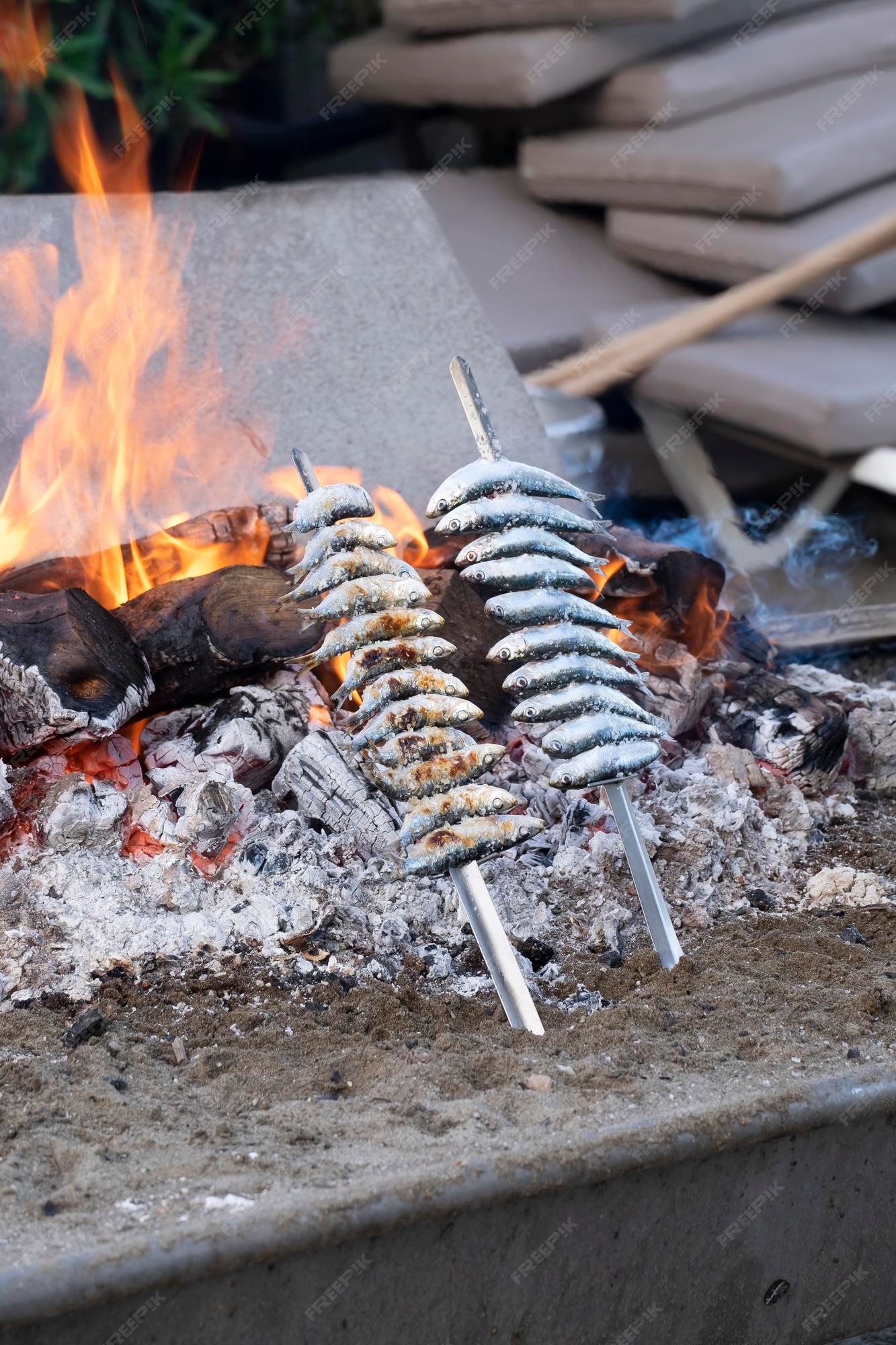In the photograph, a vivid scene unfolds of someone cooking fish over an open fire. The fire pit, made of cement, cradles glowing charcoal briquettes, some of which have turned to white ash, while others retain their blackened look. Licking orange flames reach upwards, adding intensity to the scene. Two silver metal skewers, each with 8-10 small fish resembling sardines or minnows, are propped up within the pit. The skewers are stuck at an angle, embedding their tips into the ash or sand to lean over the flames. The right skewer has been turned, revealing fish that are already browned and cooking evenly, while the left skewer's fish remain untouched by heat, looking fresh. In the background, just to the right, tan chair cushions are stacked, juxtaposing the rugged simplicity of the fire setup. A small plant is also visible, adding a touch of greenery to the otherwise earthy and fiery composition.